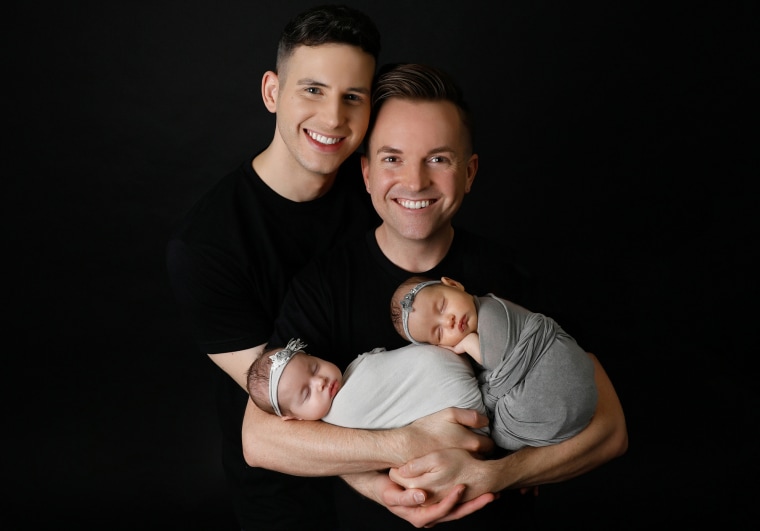This is a highly detailed family photograph set against a solid black background, creating a striking contrast. The image captures two men with light skin and short, dark brown hair, both beaming with big, bright smiles, emphasizing their happiness. They are wearing black t-shirts that blend seamlessly into the black background, making their heads appear almost disembodied. The men are a loving couple, and they are tenderly holding twin baby girls.

The twins are peacefully asleep, cradled securely in the men’s intertwined arms. One baby, swaddled in a gray blanket, wears a matching gray headband, her little hand resting adorably under her cheek. The other baby is wrapped in a white blanket with a white headband, adding to their angelic appearance. Their delicate, thin hair peeks out under the headbands, showcasing their tiny, patchy tufts. The men’s interconnected arms support the babies together, symbolizing a unified family bond. This image radiates warmth and joy, portraying a heartfelt family portrait with an intimate, loving atmosphere.